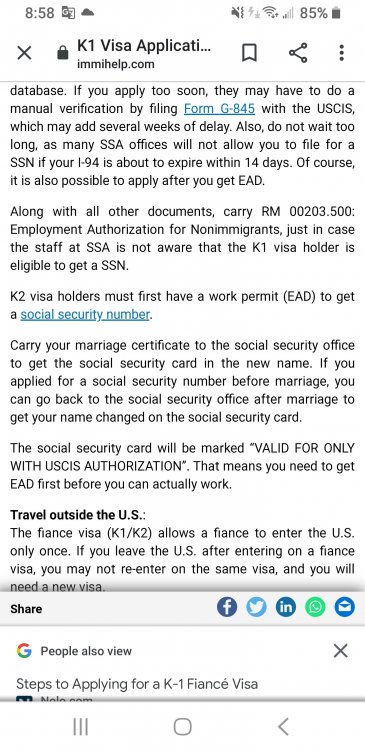This detailed caption describes a smartphone screenshot of a webpage from immihelp.com containing information on K-1 visa applications. The screenshot features content on a white background with black text and a label "858" in the top left corner. The text outlines important details and steps related to K-1 and K-2 visas:

- Caution against applying for a visa too soon, as it may result in a manual verification process through the filing of form G-845 with USCIS, potentially adding several weeks of delay.
- Advice to not delay the application excessively because many Social Security Administration (SSA) offices may not permit filing for a Social Security Number (SSN) if the applicant's I-94 form is set to expire within 14 days.
- Information that SSN applications can also be submitted after obtaining Employment Authorization (EAD).
- Instructions to carry document RM00203.500 titled "Employment Authorization for Non-Immigrants" to SSA offices, in case staff are unaware that K-1 visa holders are eligible for an SSN.
- Requirement for K-2 visa holders to obtain a work permit (EAD) prior to getting an SSN.
- Advice to bring a marriage certificate to the Social Security Office (SSO) to update the SSN to the new name after marriage. Applicants who had originally applied for an SSN before marriage can return to SSO to change their name on the SSN card post-marriage.
- Information on SSN cards being marked "valid for work only with USCIS authorization," necessitating EAD before lawful employment.
- Travel restrictions under K-1/K-2 visas, emphasizing that they allow one-time entry to the U.S., and re-entry on the same visa is not possible if the visa holder leaves the U.S.; a new visa will be required for re-entry.

The webpage serves as a comprehensive guide for K-1 and K-2 visa applicants navigating the complexities of acquiring and using an SSN, along with important travel considerations.